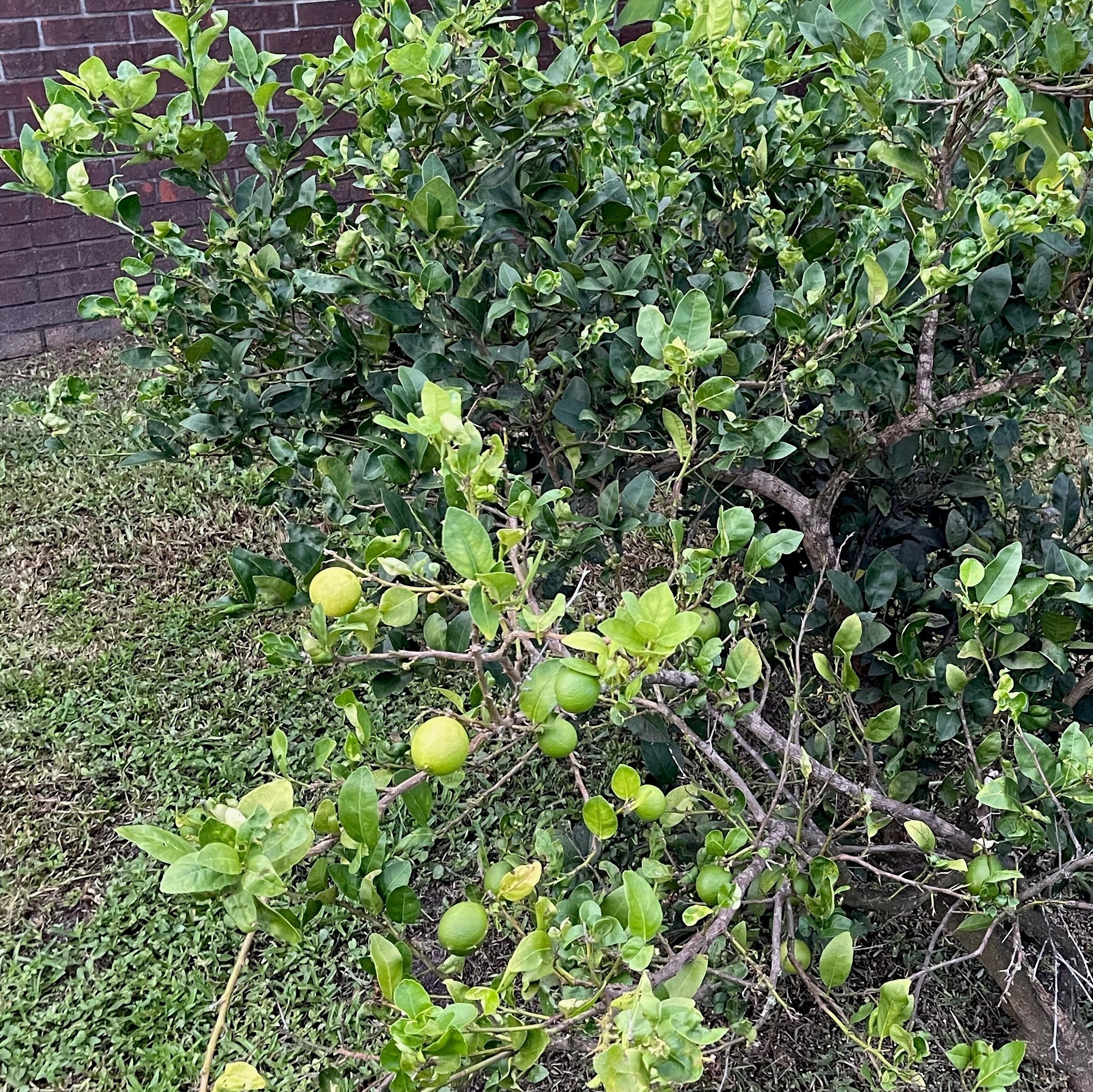This color photograph captures a garden in a yard with a distinctly detailed backdrop and well-defined elements. The background features a weathered red brick wall with white grout, partially covered by a large, dark green-leaved shrubbery. The bottom section of the image shows a neatly trimmed green grass lawn. Dominating the foreground is a small, possibly dwarf citrus tree, adorned with round, yellowish-green fruits that taper slightly at the ends—suggestive of either lemons or limes. The tree's branches are sparsely foliated, revealing some brown branches amid the green leaves. The image, presented in a square format, uses photographic realism to depict the serene, horticultural setting with a combination of green and earthy tones.